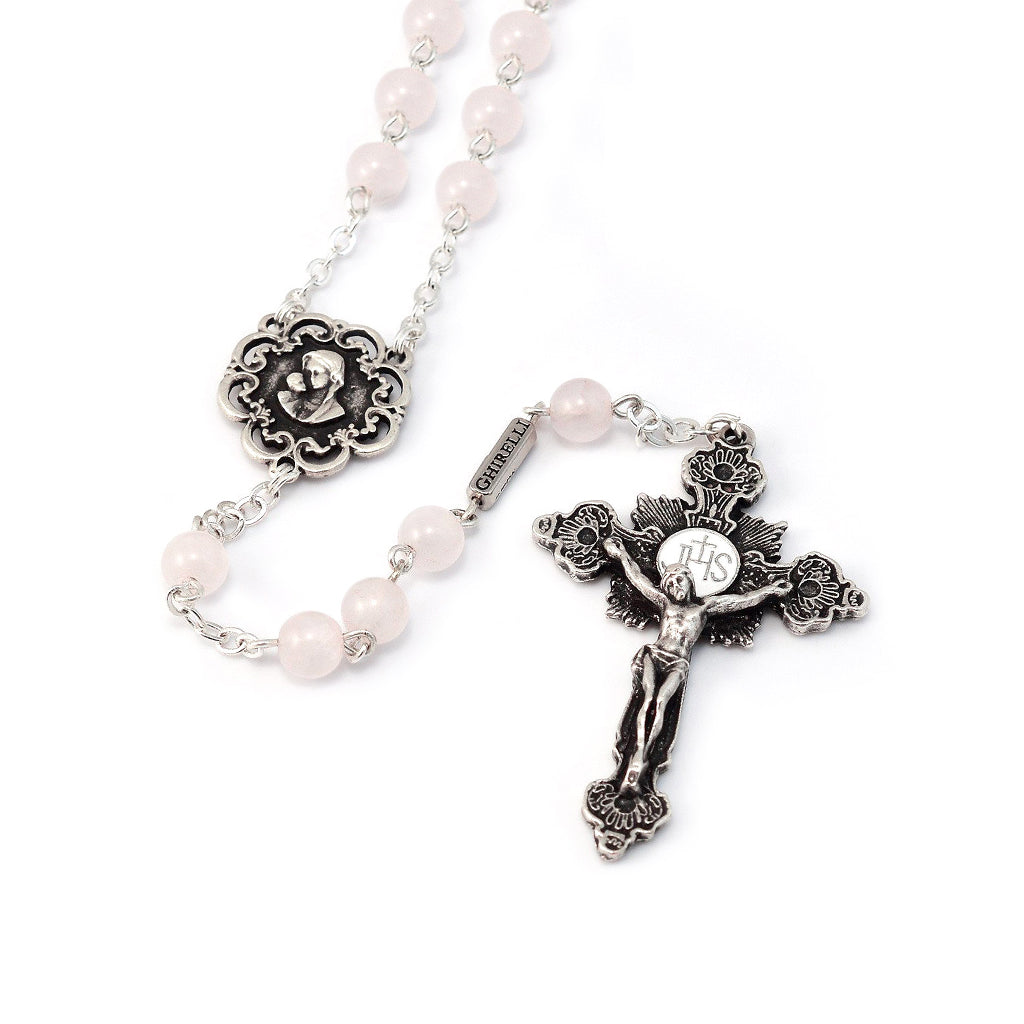The image depicts an intricate and ornate set of rosary beads, meticulously designed with precious materials. The central feature at the base is a detailed silver crucifix, showcasing Jesus on the cross, adorned with artistic flourishes. Attached to the crucifix is a series of pearls interlinked by delicate silver chains. Along the chain, a small charm bears the name G-H-I-R-E-L-L-I, 'Ghirelli', adding a distinct label to the piece. Ascending the chain, the beads culminate in a circular medallion featuring an elegant depiction of the Virgin Mary with baby Jesus in her arms, both framed by an elaborate swirl and scroll pattern. This medallion is accented by Mary's shawl gracefully draping over her head while she gazes down lovingly at Jesus, who looks up at her. The entire rosary, comprising pearls and silver strands, leads to a wearable necklace design, combining both devotion and artistry. This exquisite piece is set against a white background, highlighting its intricate craftsmanship and detailed embellishments.